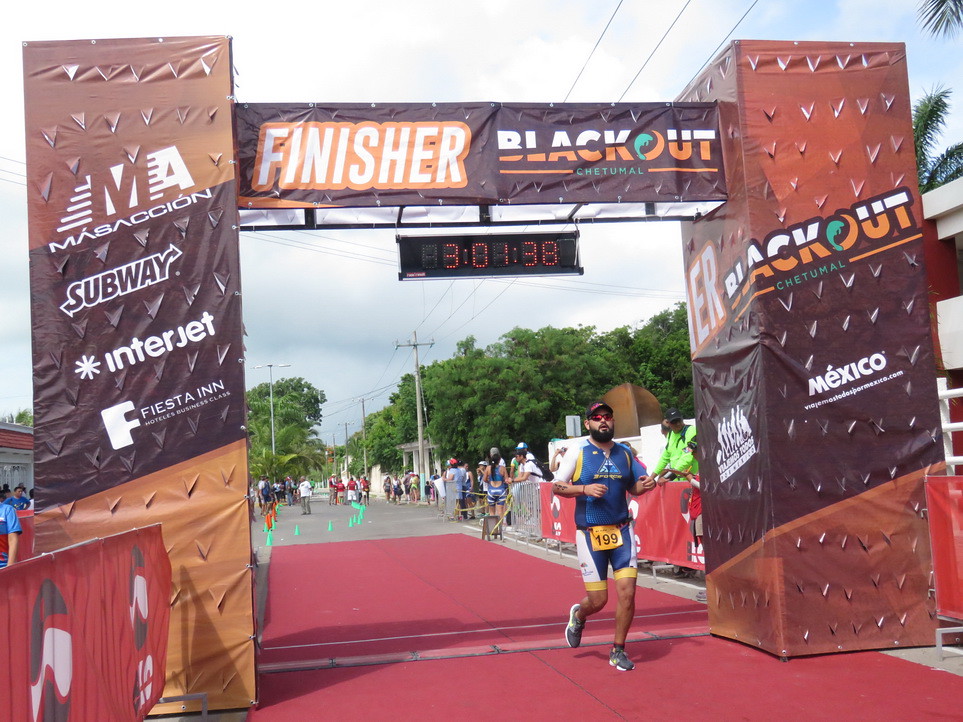A photo captures the climactic moment of a marathon as a racer crosses the finish line. The man, dressed in a full-body neoprene racing outfit that features white, yellow, and blue colors, runs determinedly toward victory. His bib number, 199, is prominently displayed on an orange sign pinned to his suit. He has facial hair and wears sunglasses, adding to his focused appearance. Overhead, a large digital clock counts up to 3:01:38, framed by the words "Finisher" and "Blackout" against the top beam of the finish line structure. This structure is supported by large columns that showcase advertisements for Subway, Interjet, Fiesta Inn, and Mexico. Below, a wide red mat guides the racers to the finish, with spectators lining the sides, and the backdrop includes trees, power lines, and a cloudy sky.